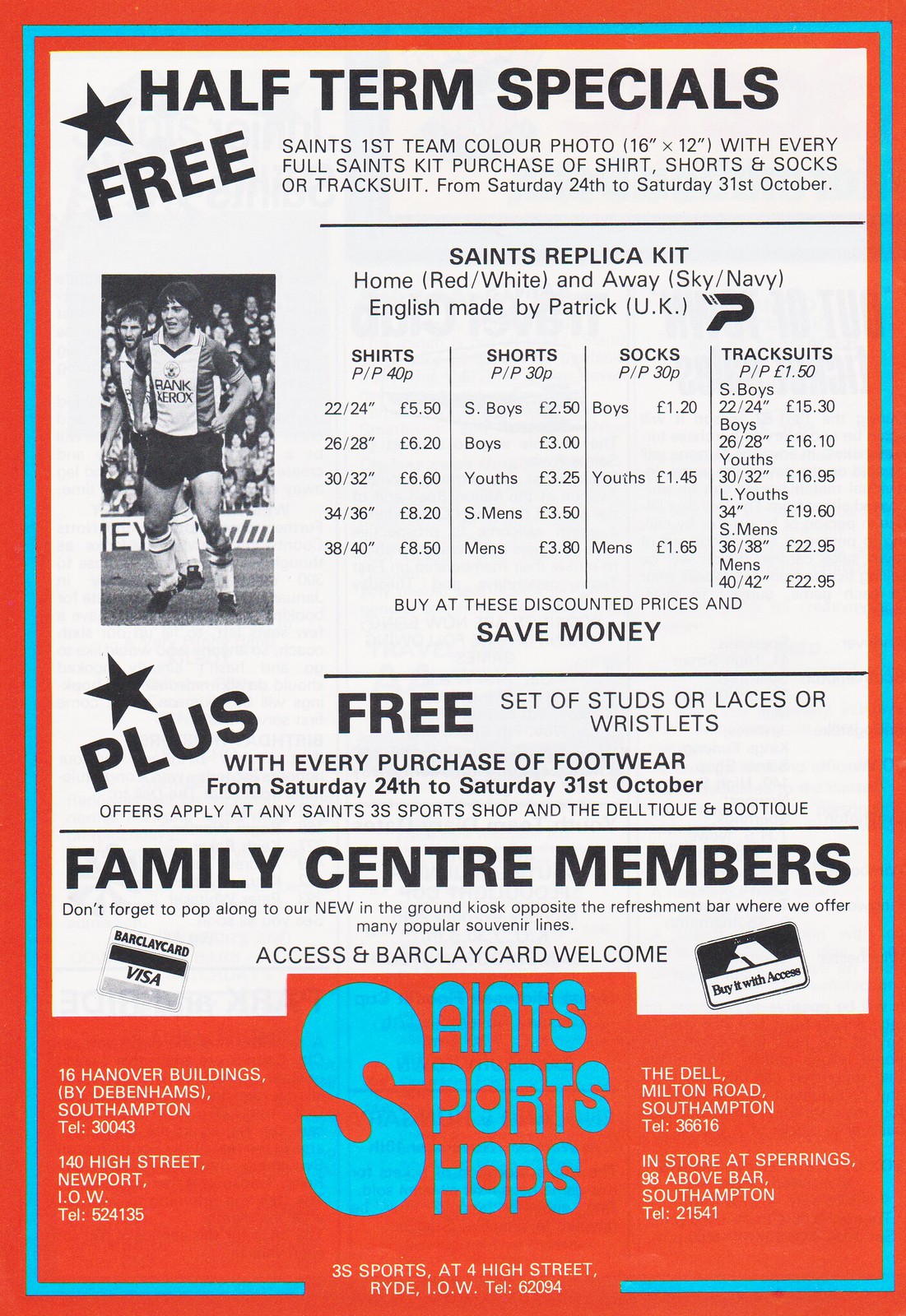The advertisement poster is quite busy but visually attractive, featuring an oblong-shaped design with a prominent orange background and a thin blue border edging around most of the poster. The main headline, "Half-Term Specials," is displayed in bold black text at the top of the poster. Underneath, there's a white section filled with black text detailing the special offers. One key feature of the promotion is a Saints First Team Color Photo, sized 16x12 inches, available with every full Saints kit purchase of a shirt, shorts, and socks, or a track suit, valid from Saturday, October 24th to Saturday, October 31st.

The poster also highlights an additional offer: a free set of studs, laces, or bracelets with any footwear purchase. The Saints Sports Shops is the name of the store, with its location in Southampton and a contact phone number, although the tiny print makes it difficult to read clearly. The bottom part of the poster, in red, emphasizes the store's name and locations, and it highlights the Saints replica kits available in home red and white or away sky and navy, made by Patrick of the UK. There are also details about the discounted prices for various items including shirts, shorts, socks, and track suits, aiming to appeal to customers looking to save money while sporting quality athletic attire.